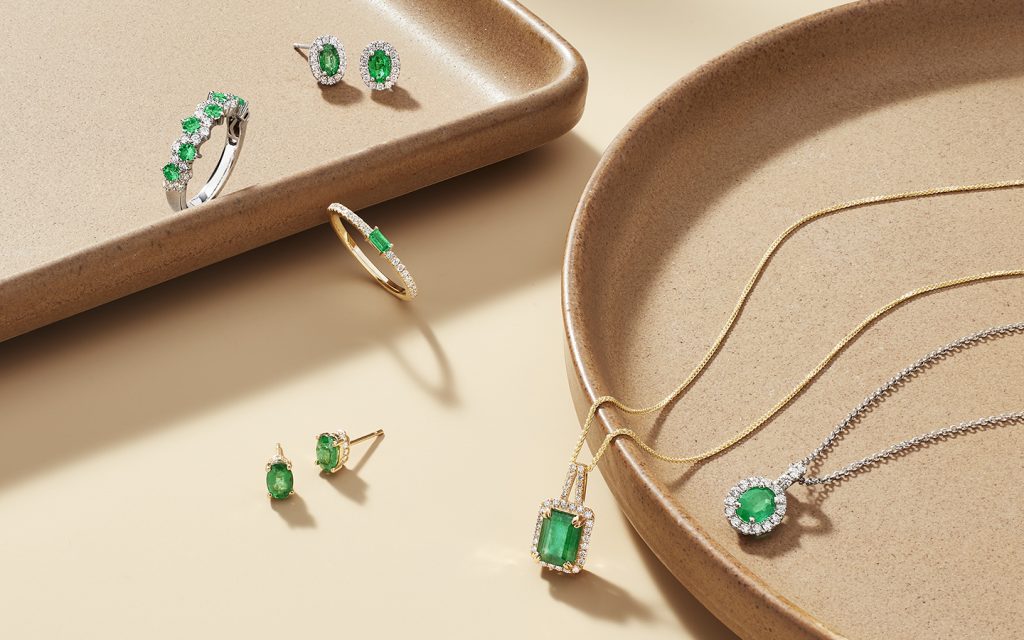The image features a tan table adorned with two trays, one square and partially cut out in the upper left corner, and a round one extending from the right towards the center. The square tray contains a silver ring with green and clear gems, and two earrings, each with a green gem and possibly diamond accents. The round tray on the right holds two necklaces; one has a silver chain with a green gem encased in a diamond-like setting, and the other features a golden chain with a similar green gem. Additionally, there are two earrings and a small bracelet with green gems and a silver outline, set on the table surface towards the bottom left. The overall display, potentially intended for an advertisement, showcases a variety of jewelry pieces including rings, earrings, pendants, and bracelets, all characterized by their prominent green stones. The trays and table surface seem to be crafted from bamboo or a similar recyclable material, contributing to a cohesive and eco-friendly aesthetic.